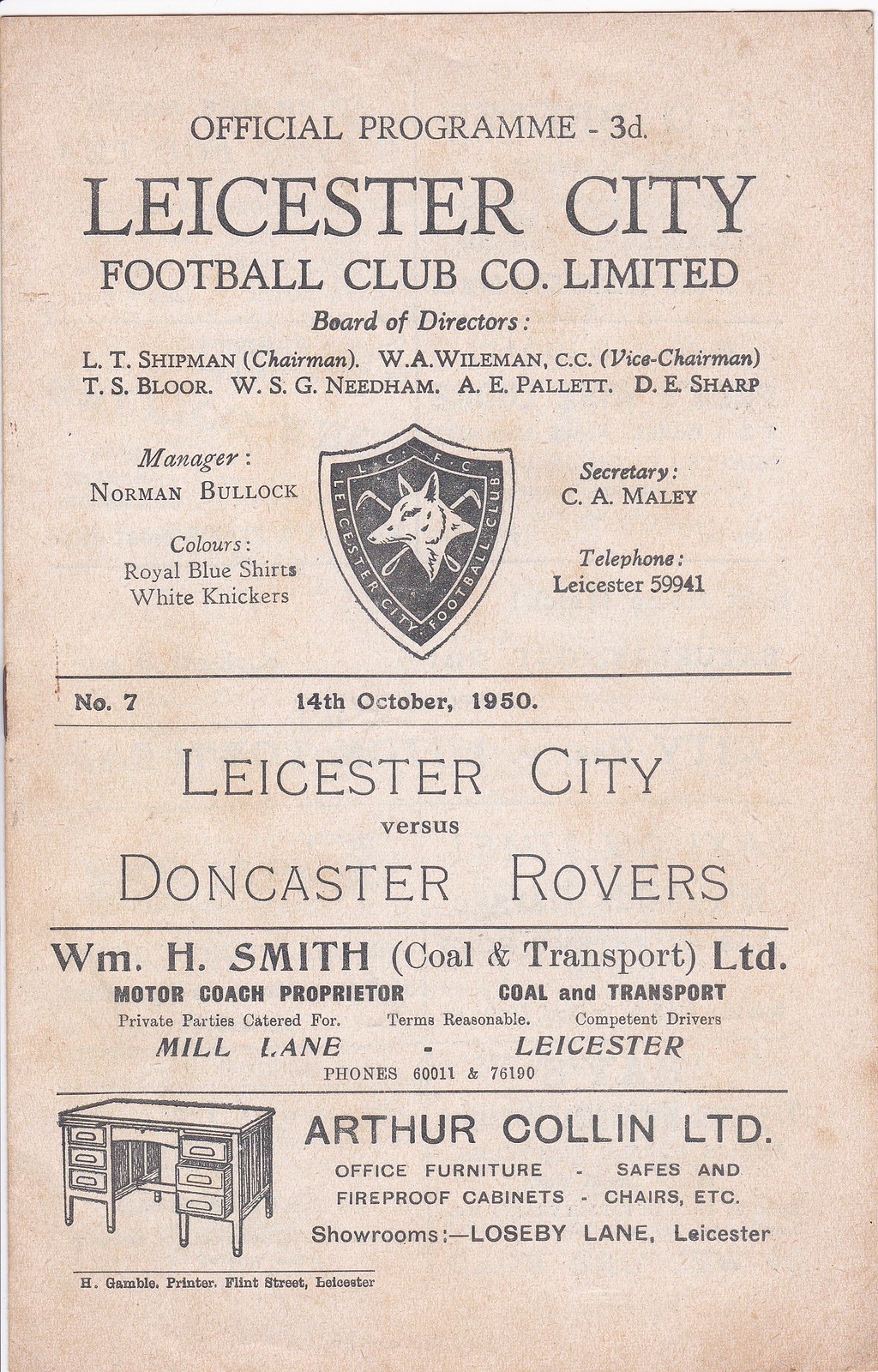The image is of an official football program from Leicester City Football Club, dated 14th October 1950. The program’s background is a faded, dirty pink color with visible splotches. At the top, it reads "Official Program 3D." Below that, it states "Leicester City Football Club Company Limited - Board of Directors" and lists various names and their positions. Centrally placed within this list of names is a distinctive shield bearing a wolf's head and the text "Leicester City Football Club."

Beneath the header, the program notes the match details: "Leicester City versus Doncaster Rovers," followed by the date, 14 October 1950, with "number 7" next to it. A thin, now-gray line demarcates this section from the advertisements below. Listed among the sponsors are "W.M.H. Smith, Coal and Transport Limited," described as a motor coach proprietor and coal transporter, and "Arthur Cullen Limited," a business specializing in office furniture, fireproof cabinets, safes, and chairs. The latter advertisement prominently features an illustration of a desk.